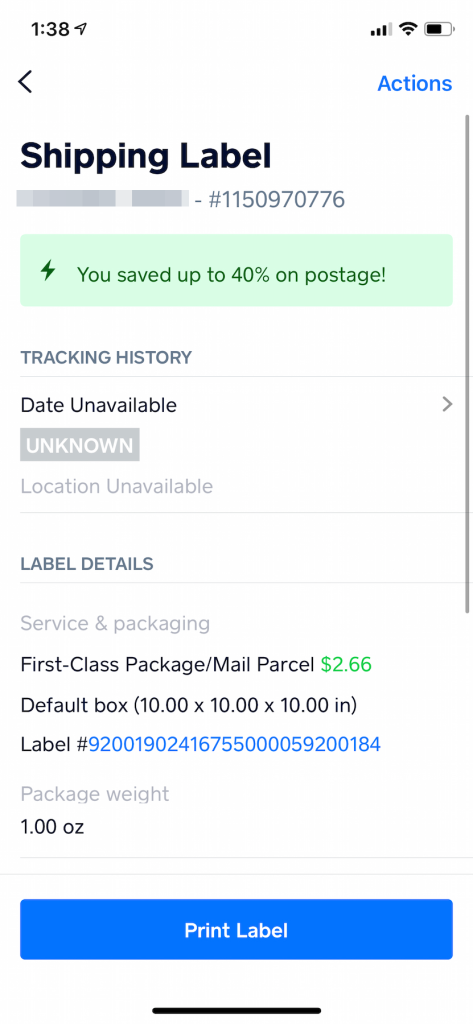Screenshot of Shipping Label in Mobile App

The image showcases a mobile app interface, specifically a shipping label within the app. The timestamp in the upper left corner reads 1:38, with a signal strength indicator showing three to four bars and a Wi-Fi signal strength at approximately 70%. The phone's battery level is also at about 70%. 

At the top of the screen, there is a back arrow on the left and a blue "Actions" link on the right. Directly below, the header "Shipping Label" is displayed, with the first two fields grayed out, followed by a reference number: #1150970776. Below this, a green banner with a lightning bolt icon announces in dark green text, "You saved up to 40% on postage!"

Further down, the section titled "Tracking History" indicates that the date, location, and other details are unavailable, suggesting this might be a mock-up or a test scenario. The "Label Details" section provides more specific information:
- **Service and Packaging:** First Class Package, Parcel Mail
- **Cost:** $2.66 (displayed in light green)
- **Default Box Size:** 10 x 10 x 10 inches
- **Label Number:** 92001902416755000059200184
- **Package Weight:** 1.00 ounce

At the bottom of the screen, a large blue button with white text prompts the user to "Print Label." Despite some fields being obscured, the interface suggests that the label is ready for printing, indicating it might be a legitimate shipping label rather than just a test.